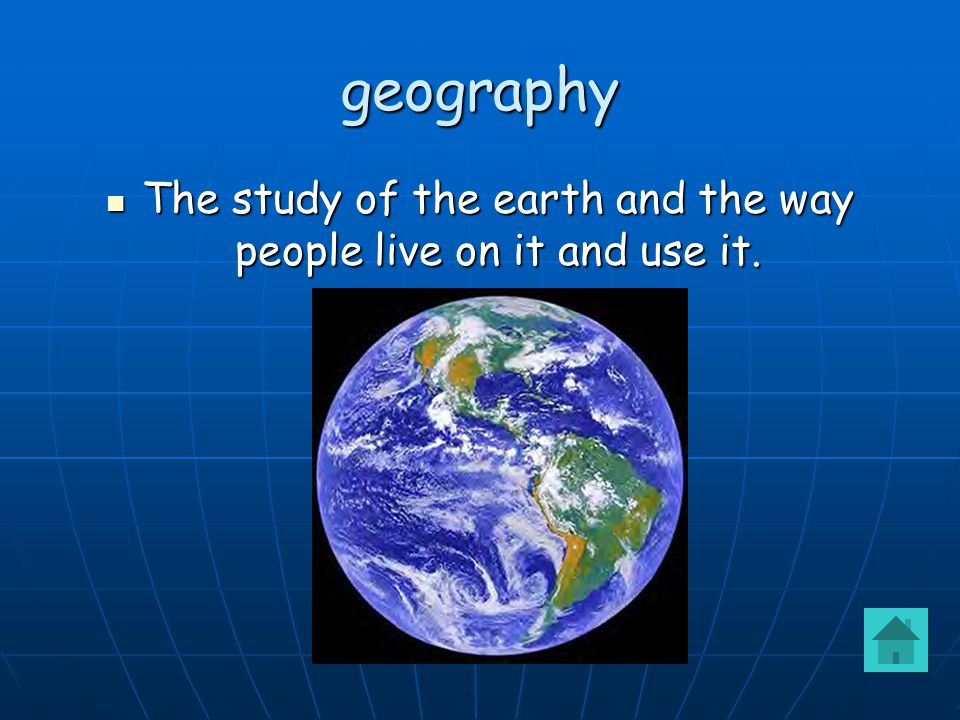The image features a definition with a visually striking design. The background is a deep blue adorned with light blue vertical and horizontal lines forming a grid, punctuated by gentle white curved lines. At the top of the image, the title "geography" is displayed in all lowercase letters, rendered in Comic Sans font with a light blue color that contrasts sharply against the darker background. Below the title, a small yellowish square serves as a bullet point, introducing the definition written in white Comic Sans text: "the study of the earth and the way people live on it and use it."

Dominating the center of the image is a realistic depiction of Earth, enclosed within a solid black square. This NASA-like view showcases the planet with vivid blue oceans streaked with white, green continents with hints of brown and orange near the edges. Finally, in the bottom right corner of the image, there is a small blue-green icon of a house with a triangular roof, adding a quaint touch to the overall composition.